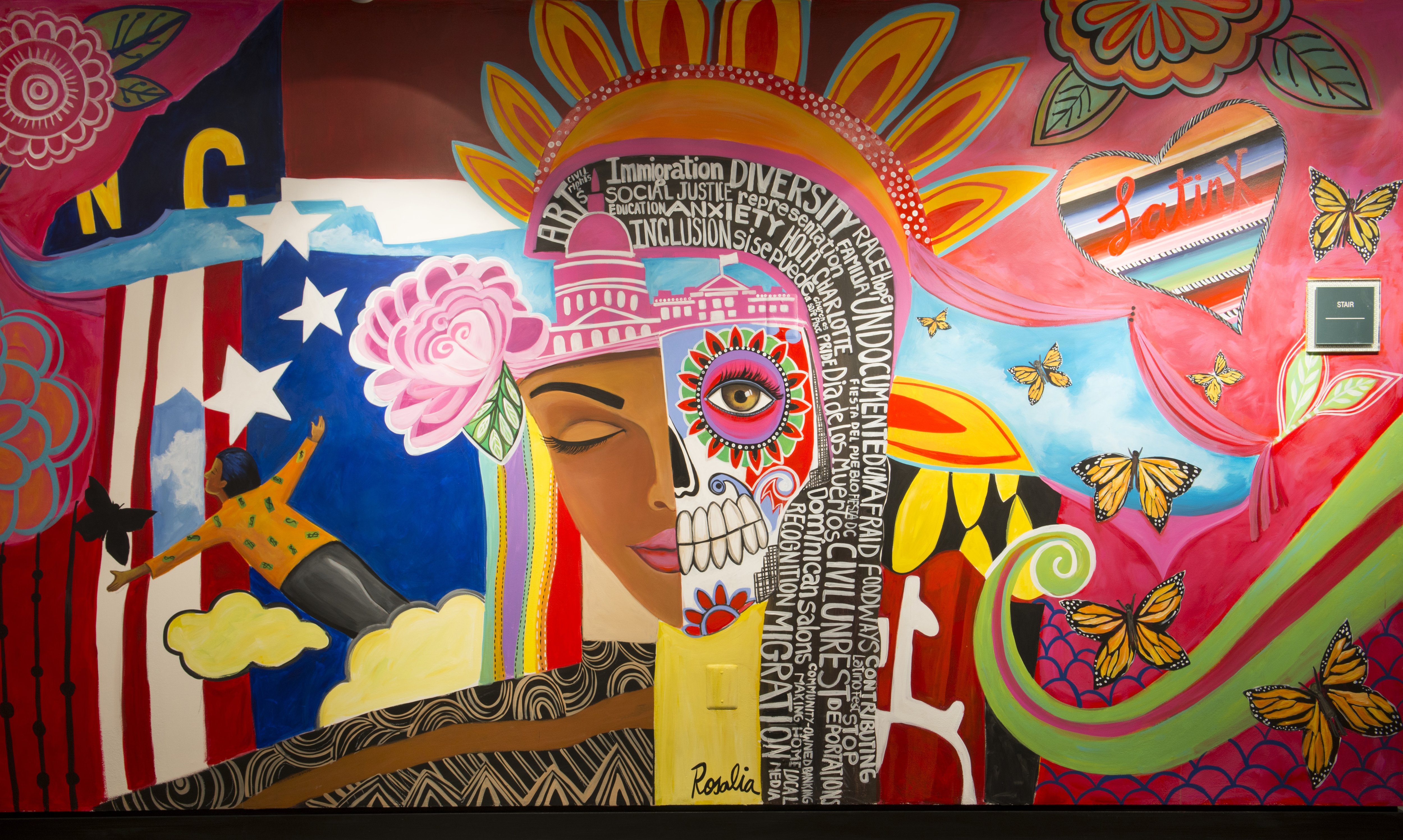This vibrant and intricate mural, possibly painted by an artist named Rosalia, centers around the face of a woman composed in a collage-like manner. The left half of her face (on the viewer's right) resembles a Día de los Muertos skull with its eye open and looking directly at the viewer, while the right half of her face is normal, featuring a closed eye and slightly downward tilt, creating a cohesive yet juxtaposed visage. The woman's hair is made up of words such as "art," "immigration," "diversity," "anxiety," "undocumented," "civil unrest," and "migration," though many are too small to read clearly. Above her hair, she dons a crown or headdress resembling a sun with orange beams extending outward.

To the left of the woman (viewer’s left), there are yellow letters "NC" and a red and white striped pattern with a person flying towards it amidst a blue sky and a black bird. The stars appear to be coming off the stripes, enhancing the dynamic aspect of the scene. On the right of the woman (viewer’s right) are numerous monarch butterflies, a green twist shape with a red stripe, and a heart adorned with multicolored stripes and the word "Latin X" written in red text, though somewhat obscured by the overlapping red stripe. Above the heart is an orange flower with two leaves, and some sections feature blue sky and yellow clouds, as well as other flowers and patterns, conveying a sense of depth and movement.

Amidst the bright and warm colors, including dominant pinks, oranges, and reds, the mural exudes a modern, lively atmosphere that merges cultural elements, symbolism, and abstract components into one cohesive, detailed artwork.